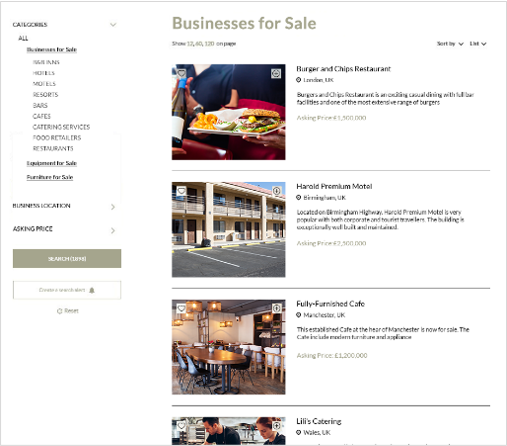The image features a website interface primarily focused on business listings available for sale. On the right side of the image, taking up the majority of the space, is a section titled "Businesses for Sale." This section includes several detailed listings of various businesses available for purchase. Specifically, there are listings for a Harold Premium Motel, a Fully Furnished Cafe, and a Burgers and Chips Restaurant, among others. 

On the left side of the image, there is a vertical menu labeled "Categories" at the top. Directly below "Categories," the menu is sorted under "All," which is highlighted. Further down, the menu lists nine distinct categories of businesses for sale, though the specifics are somewhat hard to read. Among these potential categories are cafes, catering services, food retailers, restaurants, resorts, and hotels. Additionally, there is an "Asking Price" option displayed beneath the business listings on the right side.

The interface is designed to facilitate the search for business opportunities, providing a comprehensive view of available options alongside a navigable category menu for easier filtering.